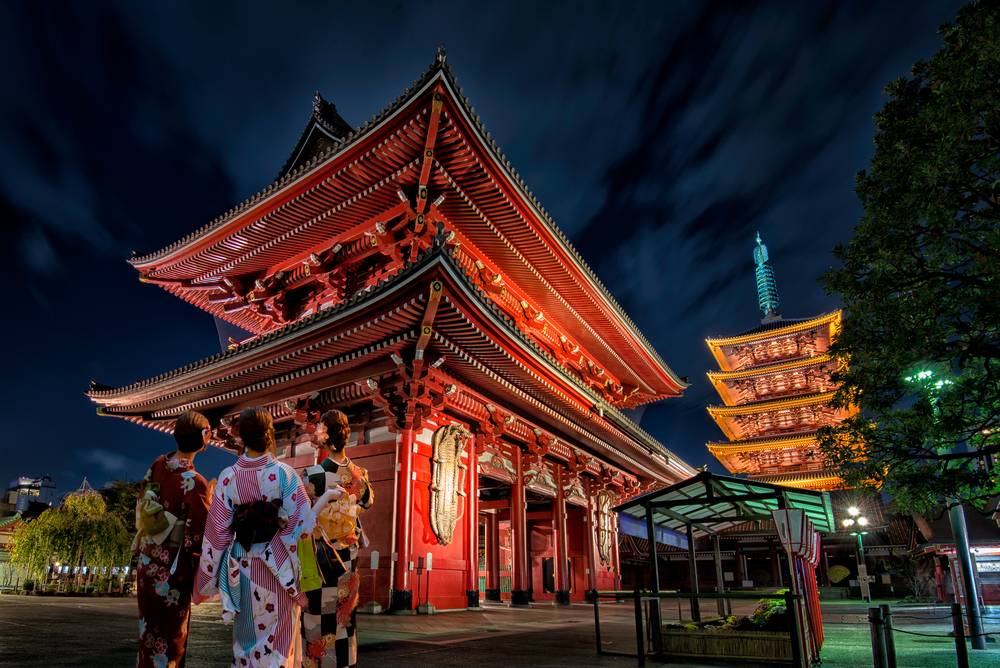This photograph captures a beautifully lit nighttime scene of a traditional East Asian temple complex, featuring prominently a striking red Chinese temple with layered rooftops in the foreground. The building is illuminated, showcasing its architectural details against the dark, deep blue night sky which is sparsely dotted with clouds. In the frame's bottom left corner, three women stand with their backs to the camera, gazing at the temple. They are dressed in vibrant traditional attire, with one wearing a maroon outfit, another in a pink and light blue ensemble, and the third in a black and white checkered garment. To the right of the red temple, another yellow temple is visible, also brightly lit, enhancing the scene's enchanting atmosphere. The surrounding area is adorned with trees, contributing to a serene and culturally rich ambiance. In the bottom right corner, a small structure glows with green light, adding another layer of visual interest to the photograph.